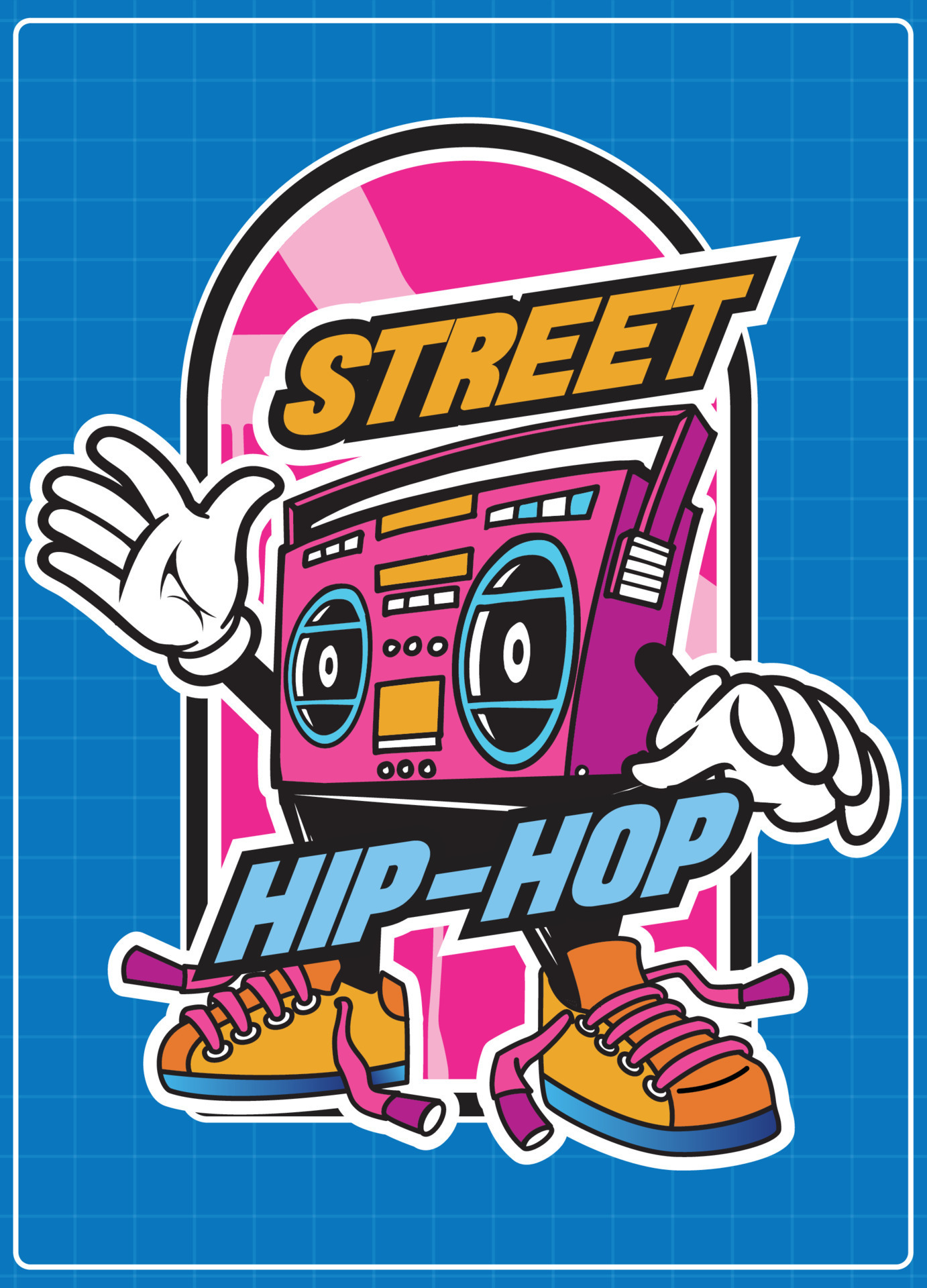This image presents a vibrant, retro-inspired graphic design set against a blue gridded background reminiscent of graph paper, complete with a clean white border arranged in portrait orientation. At the center, a black and white bordered archway houses a character depicted as a lively, anthropomorphized boombox. The boombox, which serves as the character’s head, features a distinctive pink handle and face, with blue-detailed speaker grills designed to resemble expressive eyes. 

Accentuating the playful persona, the speakers have blue vertical lines suggesting eyelids with white neodymium drivers as pupils, adding to the cartoonish charm. Positioned below the tape slot, functioning as the nose, the word "hip hop" stands out in light blue font, partially overlaying the character’s black legs. This boombox character sports bright yellow sneakers with pink laces and blue soles, evoking a sense of dynamic movement. The left hand, featuring a white glove, extends outward in a friendly wave, reminiscent of classic cartoon characters.

Above the boombox character’s head, the word "street" is prominently displayed in bold yellow lettering, enhancing the funky and fresh aesthetic of the image. The overall effect is a nostalgic nod to the 80s era, combining elements of street culture and retro design with a modern cartoonish twist, making for an eye-catching and lively visual.